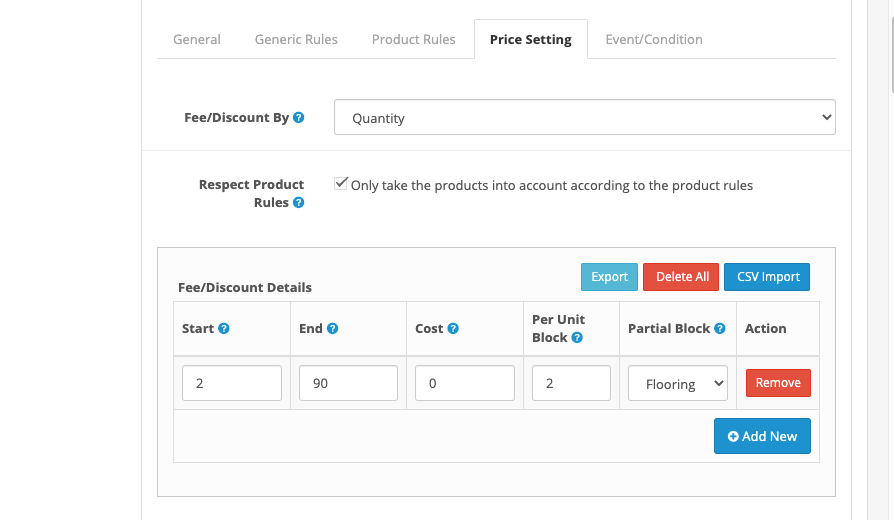Screenshot of a business software interface captured from a non-mobile device, such as a tablet, laptop, or desktop. The interface primarily features a white background with black text. At the very top, there are five category tabs labeled as: General, Generic Rules, Product Rules, Price Setting (highlighted in bold, indicating it is the current tab), and Event/Condition.

Below these tabs, there is a heading "Fee/Discount Buy" accompanied by a blue question mark icon, likely offering more information upon interaction. Directly below this heading, there's a drop-down menu labeled "Quantity," though its contents are not visible.

Further down, the section titled "Respect Product Rules" also features a blue question mark icon for additional details. This section includes a checked checkbox labeled "Only take the products into account according to the product rules."

The next section, titled "Fee/Discount Details," is a structured table with three action buttons on the right: a blue "Export" button, a red "Delete All" button, and a darker blue "CSV Import" button. The table headers from left to right are: Start, End, Cost, Per Unit Block, Partial Block, and Action, each accompanied by a blue question mark icon for more details.

Within the table, the following data is displayed in corresponding text boxes from left to right: "2," "90," "0," "2," "flooring." Each row ends with a red "Remove" button on the right. Below this data entry, there is a blue "Add Now" button with a plus sign icon. This interface seems to be part of a data management system tailored for business operations, focusing on price settings and discount management.